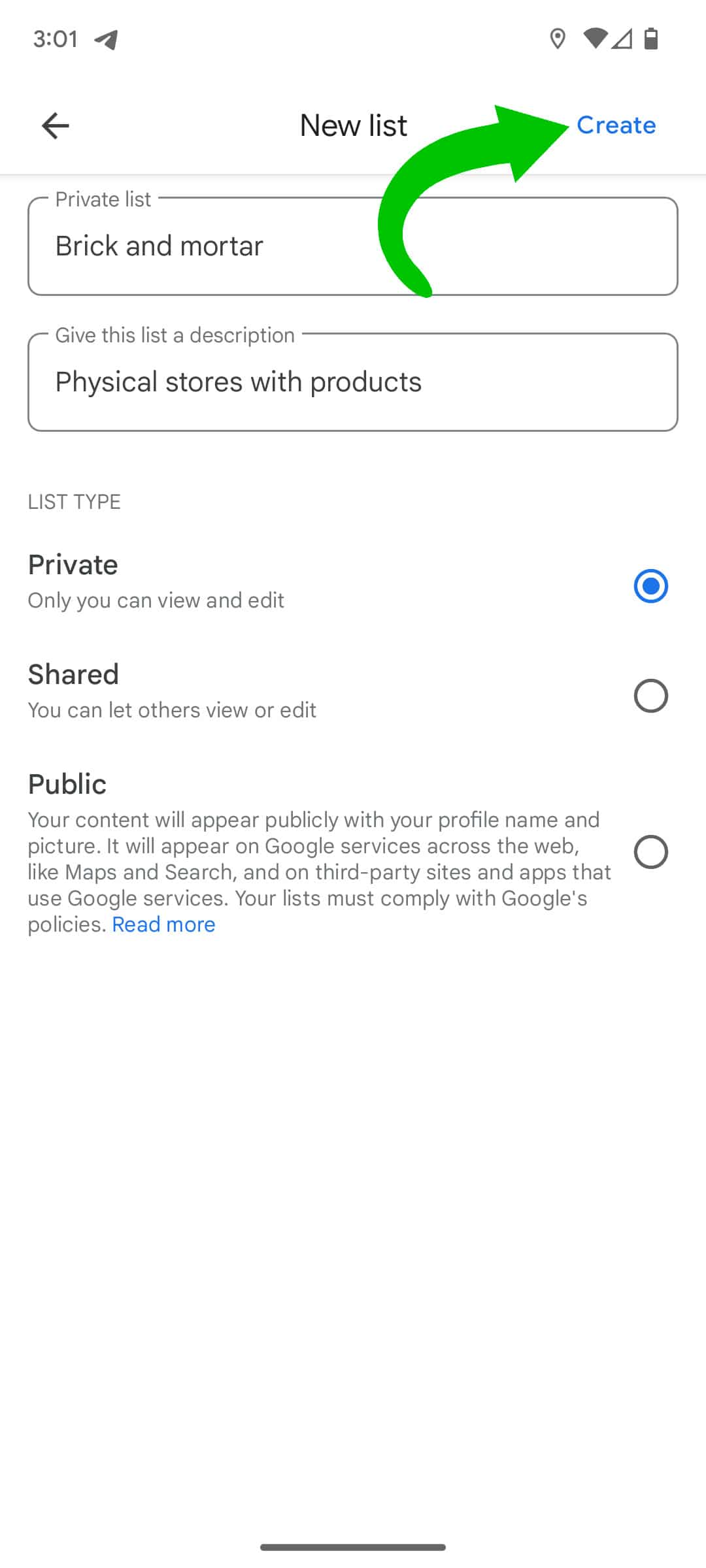This image is a detailed screenshot of a smartphone display at 3:01 PM. In the upper right corner, next to the time, there are four status icons indicating various functions: the Internet connection, battery level, and two others not specified. Below, the screen displays a page titled "New List."

On the top left, there's a back arrow, and in the top right, the option "Create" is highlighted in blue, accompanied by a prominent green arrow pointing towards it.

The main section consists of two long rectangular input bars. The first bar is labeled "Private List," with the text "Brick and Mortar" inside it, indicating the list's title. The second bar prompts to "Give this list a description" and contains the text "Physical stores of products."

Below these input bars, the "List Type" section presents three options:
1. **Private** - Highlighted with a filled blue circle, it reads "Only you can view and edit."
2. **Shared** - An unhighlighted option marked by an empty black circle, stating "You can let others view or edit."
3. **Public** - Another unhighlighted option marked by an empty black circle, explaining that "Your content will appear publicly with your profile name and picture. It will appear on Google services across the web like Maps and Search and on third-party sites and apps that use Google services." It concludes with "Your lists must comply with Google's policies," followed by a "Read More" link in blue ink.

The screenshot captures the detailed settings and options available for creating a new list on the phone screen.